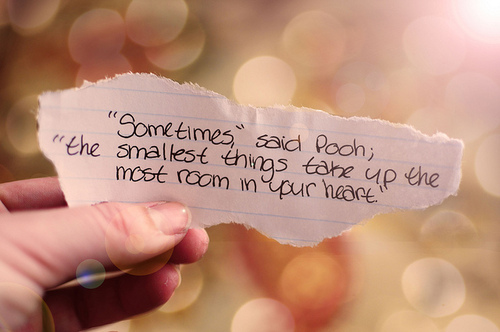In the image, a hand with long nails, likely a woman's, emerges from the left side, holding a small, torn piece of lined school paper. The paper bears a handwritten quote in a font that mimics natural handwriting, stating: "Sometimes," said Pooh; "the smallest things take up the most room in your heart." The background features a blurry, bokeh effect with starry, large, dotted patterns in shades of white, yellow, gold, and orange, giving a dreamlike quality to the scene. A sun flare in the upper right corner adds to the ethereal ambiance. The overall appearance suggests a poster or a motivational graphic, ideal for printing and displaying.